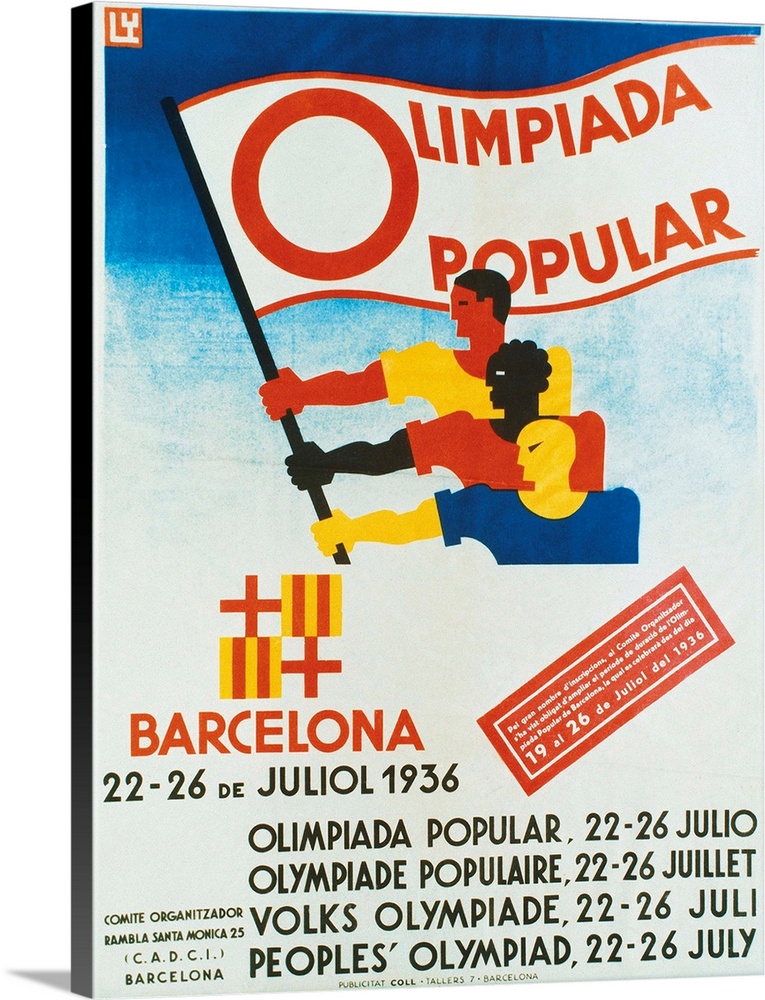This is a colorful and detailed poster promoting the People's Olympiad, scheduled to be held in Barcelona from July 22 to 26, 1936. The backdrop transitions from a deep blue at the top to a pristine white at the bottom. Prominently featured in the center of the poster are three illustrated male figures, each with distinct skin tones and appearances: one with a reddish complexion and yellow shirt, another with dark black skin and a red shirt, and the third with yellowish skin wearing a blue shirt. They are all depicted with their right arms extended upwards, clasping a flagpole. Above them, the flag waves, colored white with a red border, bearing the inscription "Olimpiada Popular." Below this central image, the text reads "Barcelona 22-26 de Julio 1936," followed by translations of "Olimpiada Popular" in various languages, including "Volks Olimpiada" and "People’s Olimpiada," accompanied by the same dates. In the bottom left corner, additional details state "Comit Organizator Rambla Santa Monica 25 CADCI," further rooting the event in its Barcelona setting.